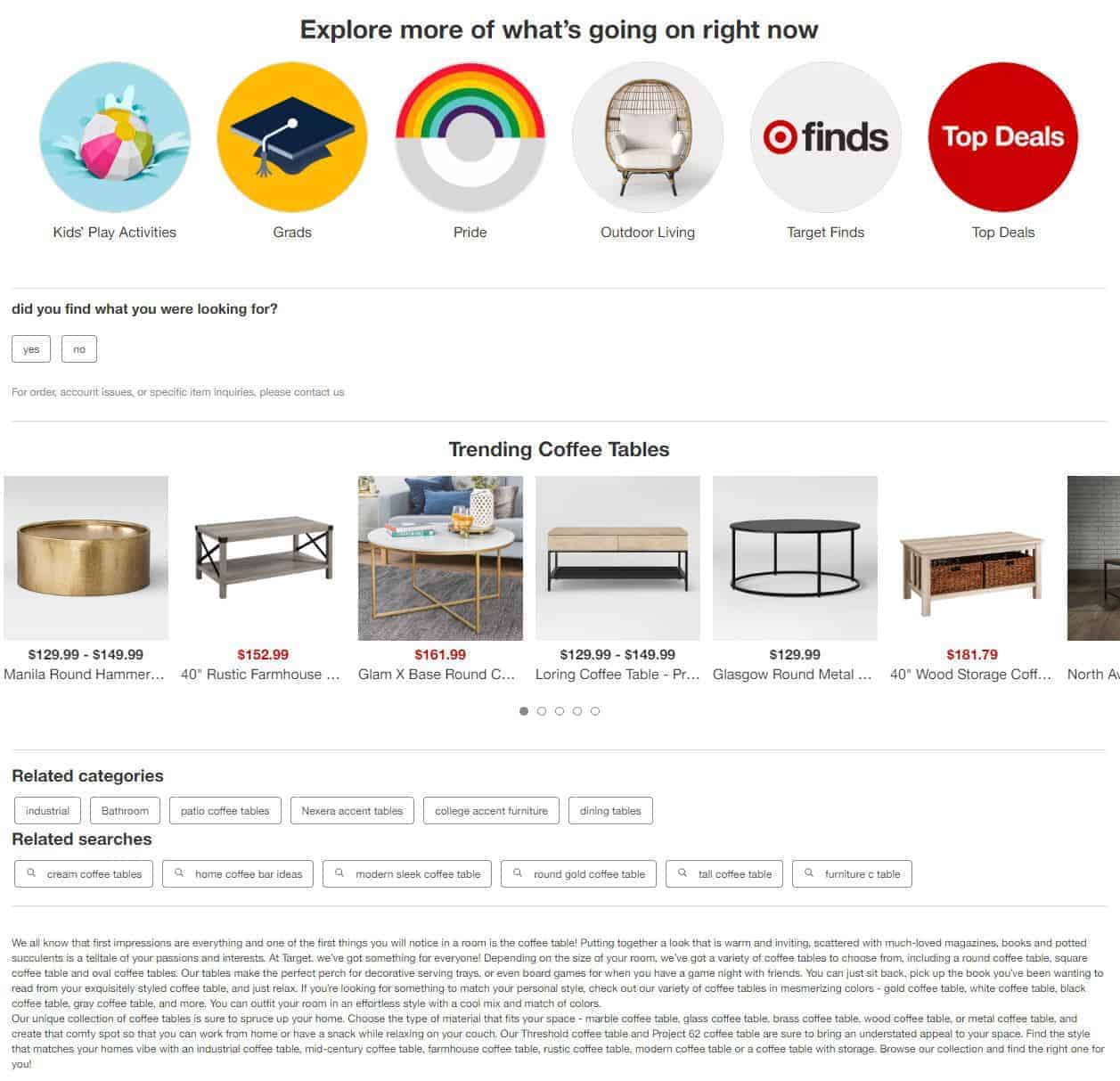The image showcases a vibrant catalog page with a clean, white background adorned with various colorful circles, each representing different categories. At the very top, bold black text invites viewers to "Explore more of what's going on right now."

- **Top Section:**
  - **Circle 1:** Features a beach ball symbolizing kids' play activities.
  - **Circle 2:** Solid yellow with a graduation cap icon, labeled "Grads."
  - **Circle 3:** Displays a rainbow on top and grey on the bottom, with the label "Pride."
  - **Circle 4:** Contains an image of a chair, signifying "Outdoor Living."
  - **Circle 5:** Labeled "Target Finds" with corresponding text below.
  - **Circle 6:** Solid red circle indicating "Top Deals" in white text.

- **Middle Section:**
  - A question asks, "Did you find everything you're looking for?" with options for "Yes" or "No" enclosed by grey lines.

- **Product Display:**
  - Shows eight images of trending coffee tables.
  - Prices are marked with red indicating sale prices and black for regular prices.

- **Bottom Section:**
  - Features additional navigation options under "Related Categories" and "Related Searches," providing various options for further exploration.